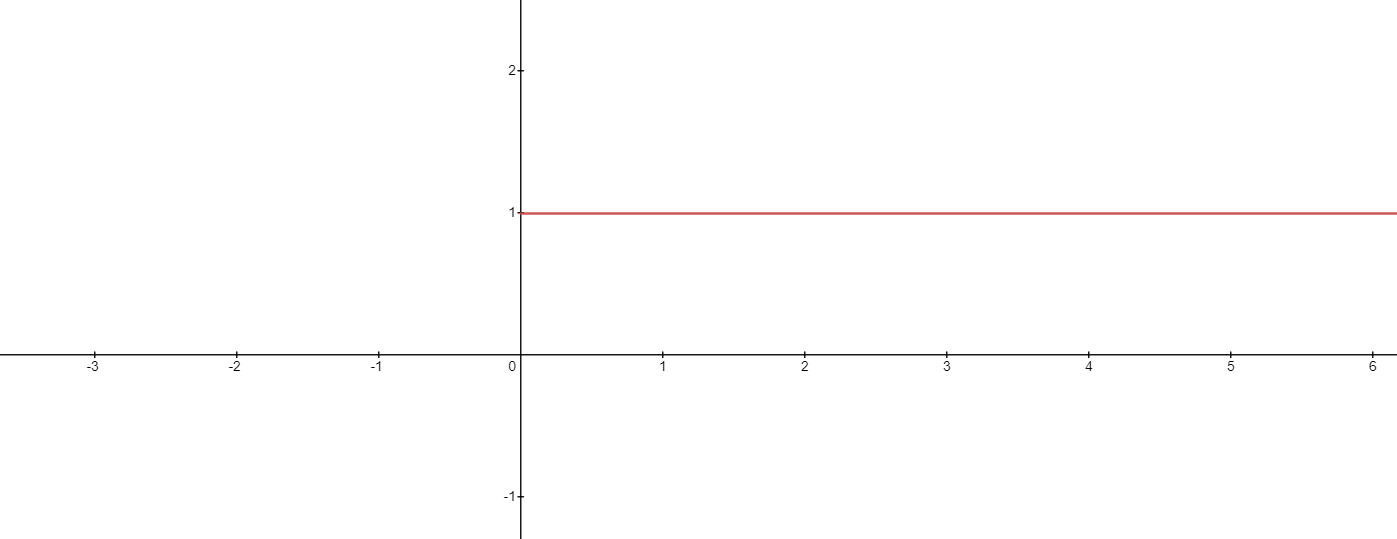The image features a simple, uncluttered graph set against a white background. It prominently displays perpendicular x- and y-axes, both in black, with the x-axis spanning from -3 to 6 and the y-axis ranging from -1 to 2. The primary focus is a thin red horizontal line that intersects the y-axis at the value of 1 and extends across the x-axis from 0 to 6. This single red line is the only graphical element depicted, emphasizing its significance in the otherwise minimalistic setting. No additional lines or text are present, apart from the numerical labels on the axes, highlighting the simplicity and clarity of the graph.